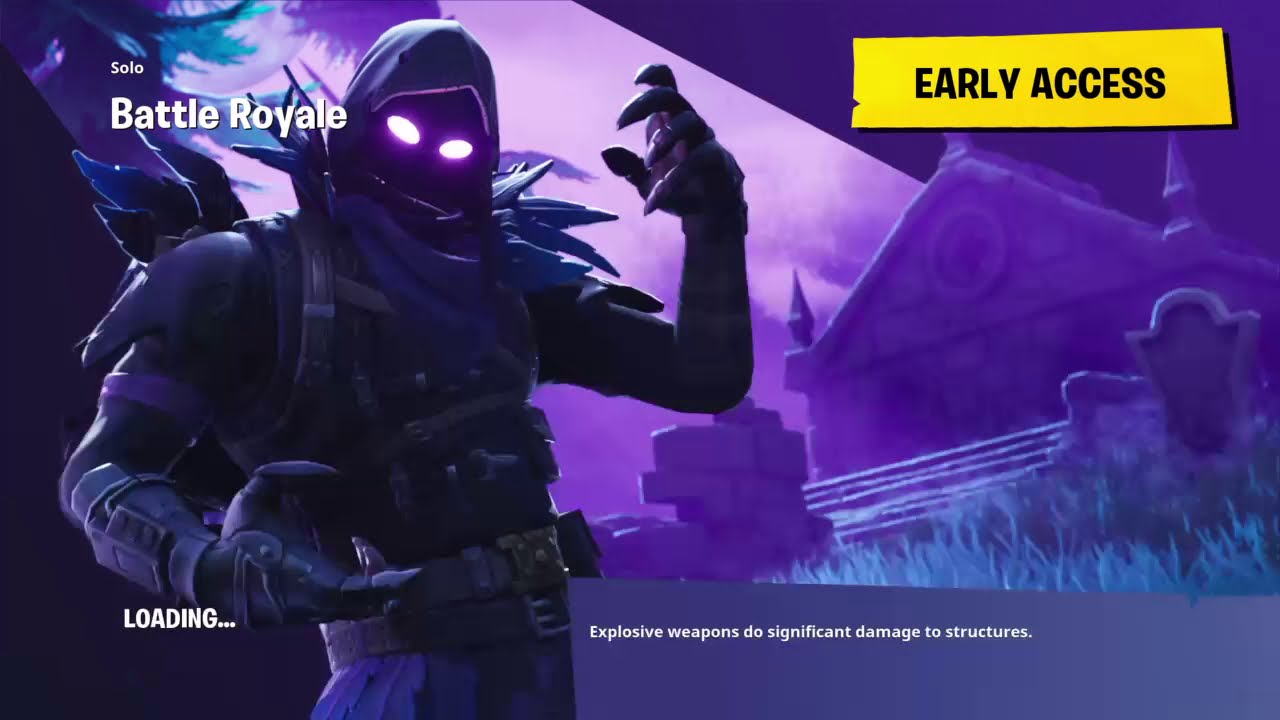The image appears to be a digital screenshot from a video game, potentially a loading screen for a battle royale style game like Fortnite or Overwatch. In the upper left-hand corner, it displays "Solo Battle Royale" in white text. The upper right-hand corner features a yellow rectangle with the words "Early Access" in black letters. The lower left-hand corner reads "Loading" in white text, while the bottom center of the screen contains a banner stating "Explosive Weapons Do Significant Damage to Structures" in white letters.

The focal point of the image is a large, menacing character positioned slightly to the left of center. The character is clad in black and purple armor, wearing a hooded cloak, and has glowing white eyes. They have an imposing presence, reminiscent of Darth Vader, with additional features like wings on their back and a collar similar to black leaves around the neck. The background is dominated by a gloomy, purple-hued cemetery scene, complete with headstones, a white fence, and structures like a mausoleum with towers and a rectangular roof. The overall environment is dark and eerie, with a purplish sky and hints of greenish-blue grass, adding to the sinister atmosphere of the image.